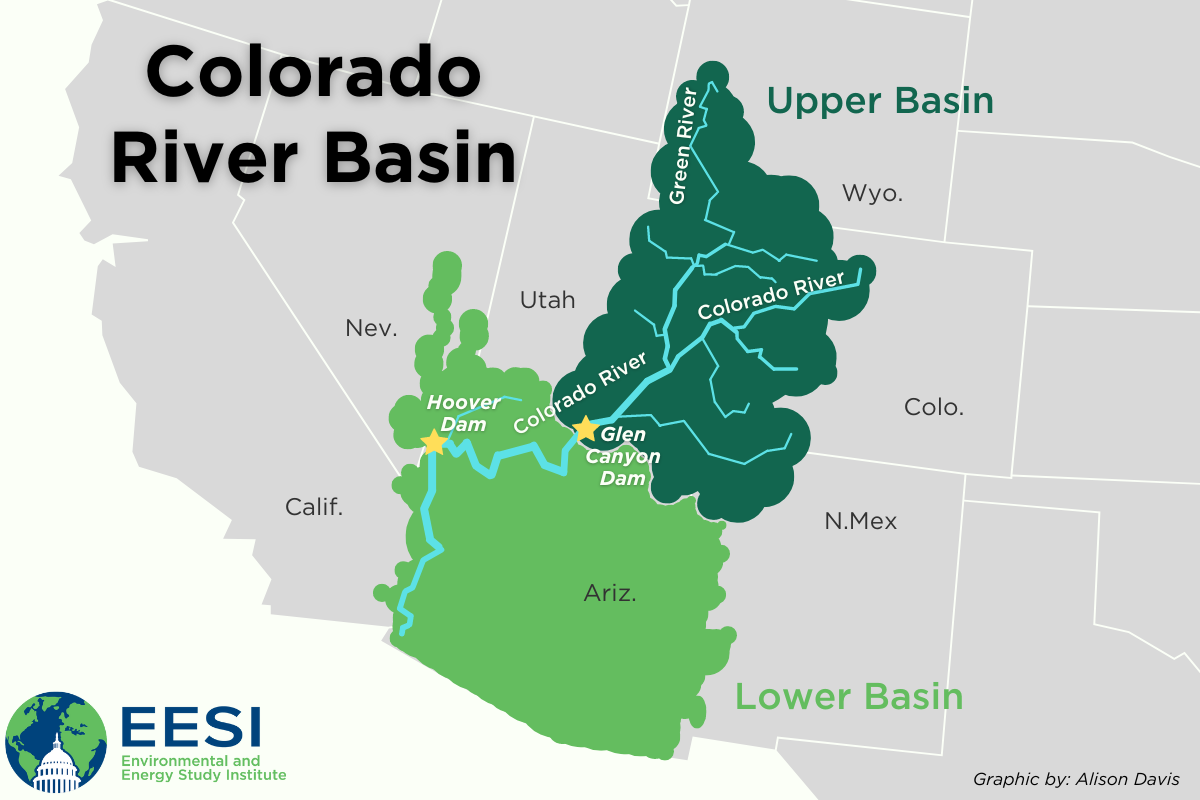This is a detailed map from the Environmental and Energy Study Institute (EESI), indicated by their logo in the bottom left corner, which features a globe with the Capitol building in front of it, accompanied by the text "EESI, Environmental and Energy Study Institute." In the lower right corner, there is a credit graphic by Allison Davis. The map prominently displays the Colorado River Basin, with "Colorado River Basin" in large black text in the top left and "Upper Basin" in green text in the top right. The map spans parts of Arizona, California, Nevada, Utah, Wyoming, Colorado, and New Mexico, and highlights the path of the Colorado River and the Green River in blue. The regions influenced by the river are marked in dark green and light green. Specific points of interest, such as the Hoover Dam and Glen Canyon Dam, are marked with stars. The map effectively illustrates the division between the Upper Basin and Lower Basin, with labeled areas highlighting the significant ecological and hydrological features in the American Southwest.